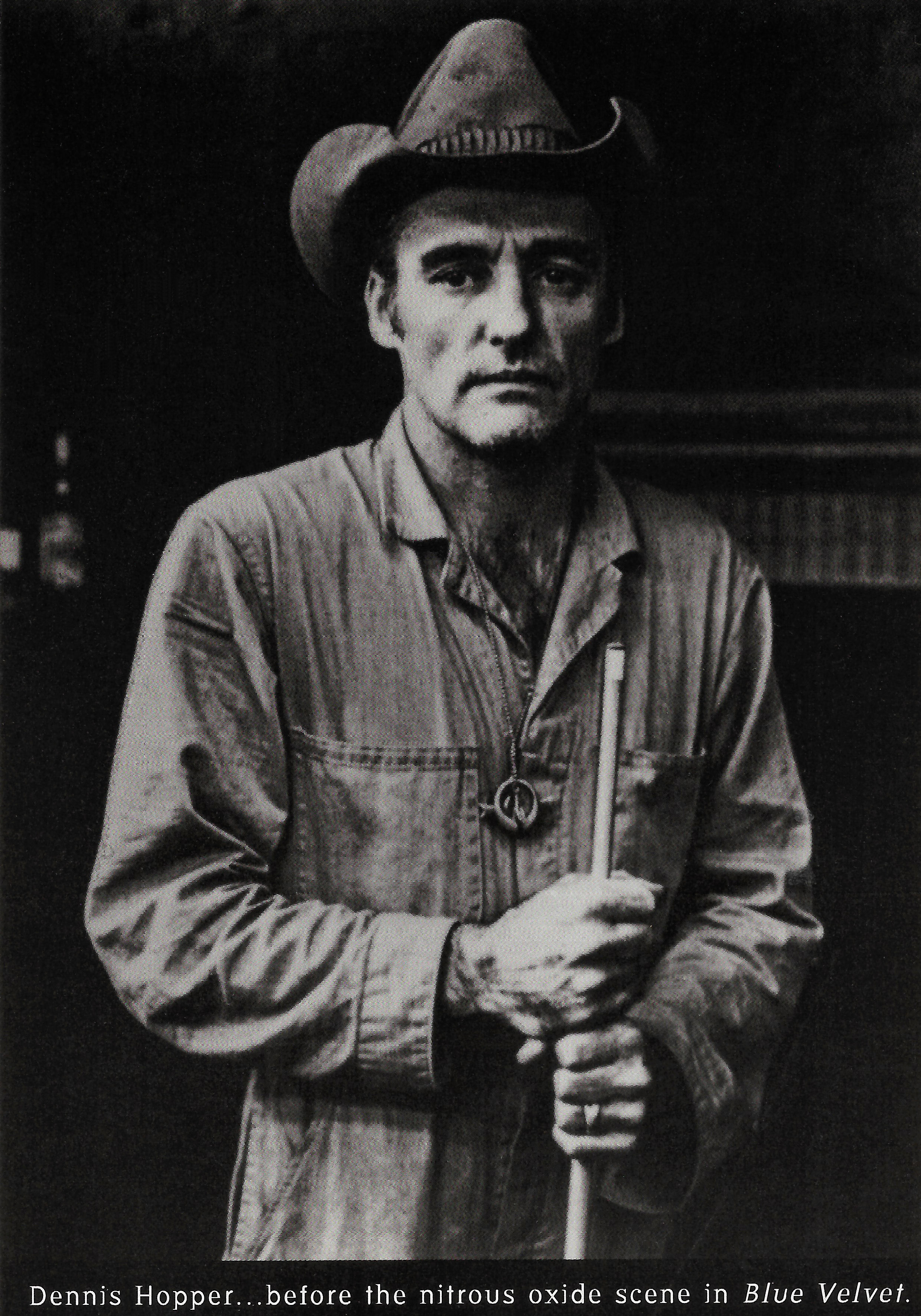This black and white photograph, reminiscent of an old magazine image, prominently features a somewhat frail-looking Dennis Hopper. Dressed in a long denim-like shirt, with pockets, he is poised solemnly, holding a stick with both hands. Hopper, clean-shaven and wearing a cowboy hat, appears introspective as he gazes directly into the camera. Adorning his left-hand ring finger is a noticeable ring, while a chain with a large dollar sign hangs around his neck. The background is predominantly dark, with faint, unrecognizable objects, possibly hinting at a building and a bottle on the left. Below the image, in white text on a black strip, is the caption: "Dennis Hopper before the nitrous oxide scene in Blue Velvet."